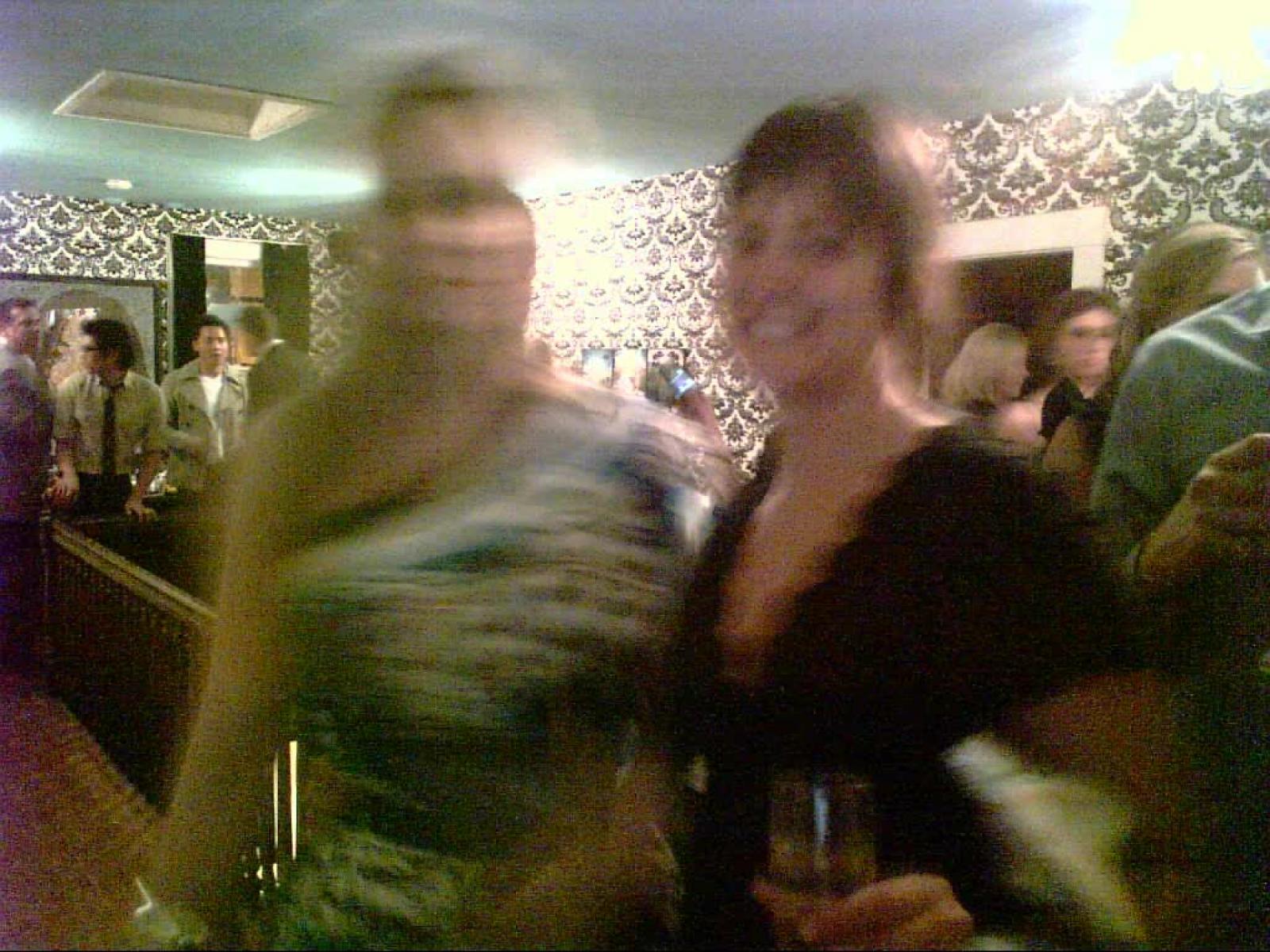In a dimly lit, indoor setting that appears to be a party or a bar, a very blurry photograph captures two women standing side-by-side as they pose for the camera. The woman on the left has blonde hair and is wearing a vibrant dress with silvers and blues that only covers her right shoulder, leaving the left shoulder bare. Despite the blur, her dress stands out. The woman beside her, slightly to the right, has short, dark brown hair and is smiling warmly. She is dressed in a low-cut black top and is holding a drink, presumably a wine glass, in her hand. Behind them, a crowd of party-goers can be seen mingling, with men and women scattered throughout the background on both sides. The wall behind them is adorned with dark, flowery patterned wallpaper, adding a touch of elegance to the lively scene. A brown, bar-like structure is visible in the background, enhancing the ambiance of the social gathering.